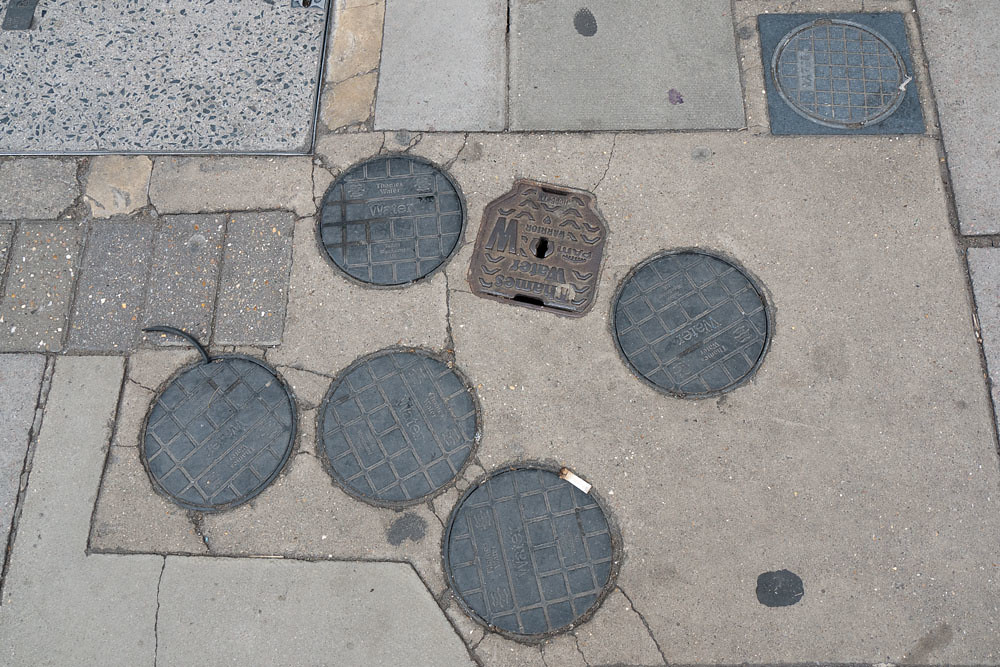This image captures a top-down view of an outdoor street or sidewalk, likely in an urban setting, featuring a diverse array of textures and details. The surface, a mosaic of variously sized and shaped concrete and granite slabs, creates a visually compelling pattern interspersed with metallic fixtures. Among these fixtures are seven manhole covers, each round with a zigzag or lattice design for grip, and a unique, rusted water sewage cover shaped like a milk carton or mug, square but tapering at the top. The color palette includes shades of blue, gray, and white with a marbled effect on the granite sections. The entire scene is accented by intricate engravings, some reading "water," and a lone cigarette butt resting on one of the covers, suggesting a well-used and aged sidewalk. Despite its complexity, the image evokes a sense of an older structure, potentially in a park, city sidewalk, or similar public area.